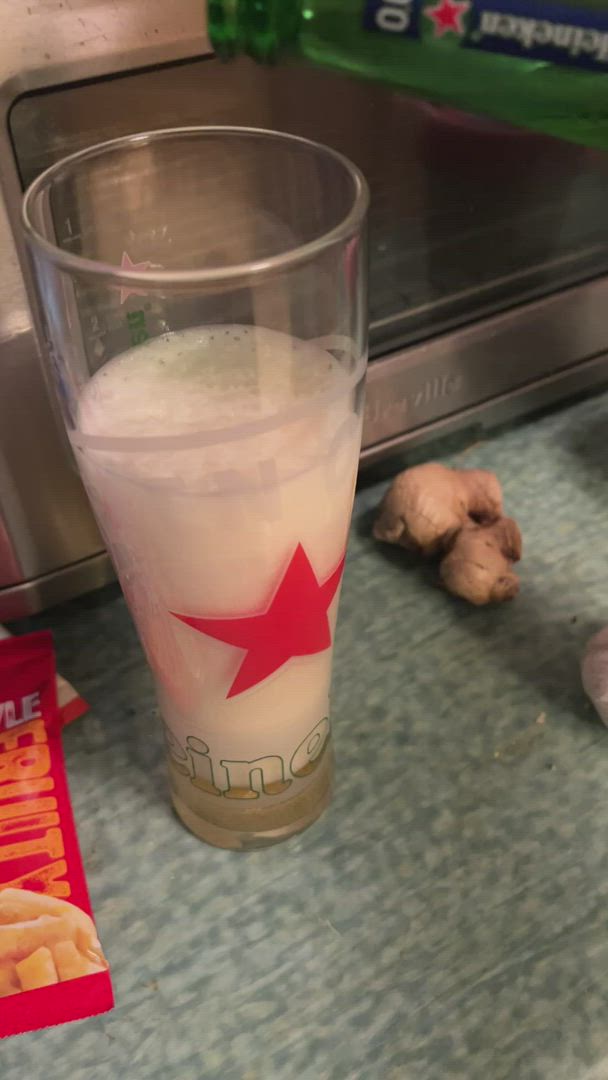This indoor photograph showcases a close-up of a Heineken beer glass filled almost entirely with white foam or milk. The glass, which is taller at the base and widens gradually towards the top, prominently features a red five-pointed star and the Heineken logo at its base. Positioned on a black tabletop with stainless steel edging, possibly a bar counter, the scene includes various elements that enhance the detailed setting: 

- In the upper right corner, an upside-down Heineken 12-pack beer box adds context, suggesting the setting may be a bar or a casual gathering place.
- To the left of the glass, a red rectangular box with yellow French fry-like pieces and yellow lettering is visible.
- A bit of a bulb of ginger is situated to the right of the glass, adding an unexpected touch to the scene.

The tabletop, appearing as a greenish or grayish bar surface, further complements the dimly lit yet focused image. What makes the photograph particularly intriguing is the unusual content of the Heineken glass, which defies expectations by being filled with foam or milk instead of the beer usually associated with the brand.